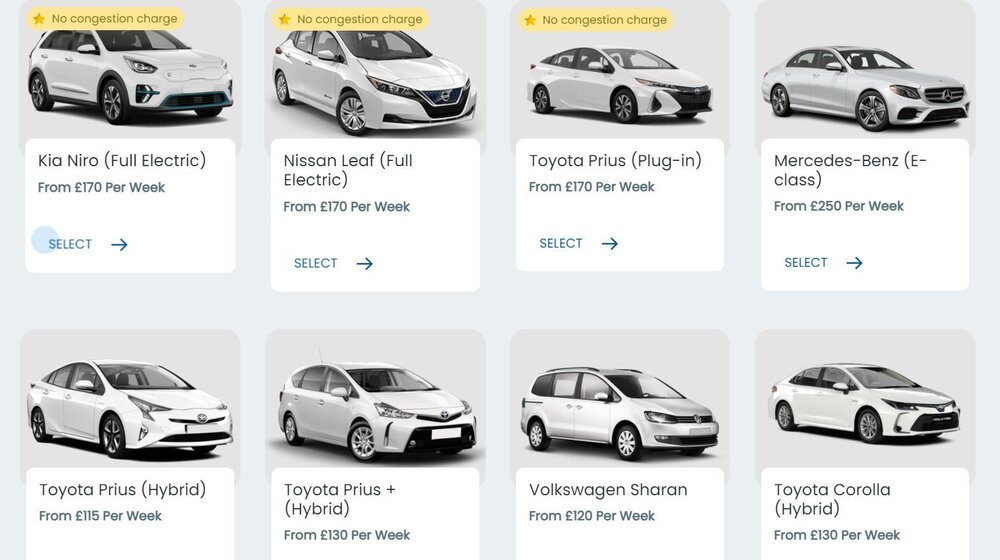A car rental search aggregator screen displays eight options matching an unseen search query. The vehicles are uniformly white, and the selection includes a diverse array of vehicle types: one SUV, one compact four-door, two sedans, three additional sedans, a hatchback, a minivan, and a hybrid sedan. Each car thumbnail is accompanied by pertinent details regarding their drivetrain: options include fully electric, plug-in electric, various hybrids, and one gasoline vehicle. This information allows potential renters to select a car that aligns with their specific requirements and preferences.